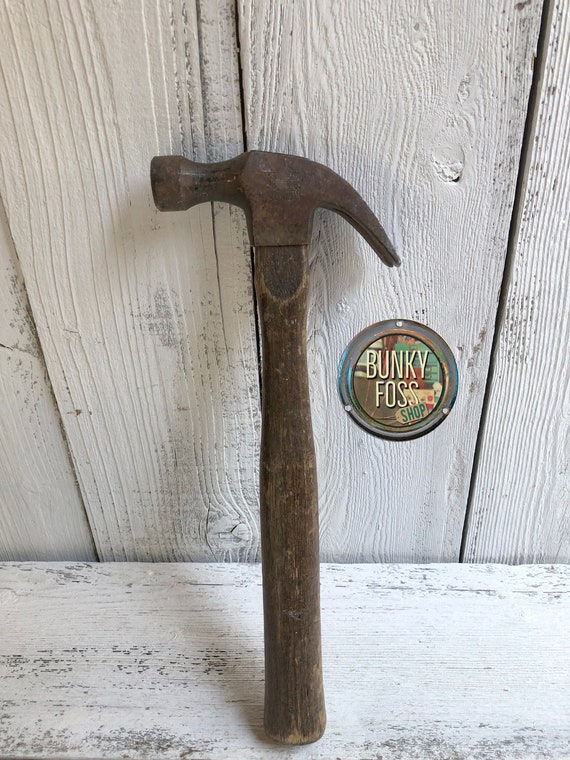The image features a vintage, upright hammer with a wooden handle and a rusted metal head, leaning against a backdrop of off-white, painted wooden planks. The paint on the planks and the floor, where the hammer is resting, appears to be peeling, enhancing the rustic and aged ambiance of the scene. To the right of the hammer is a small tag with the text "Bunky Foss Shop Below," cleverly playing on the phrase "Funky Boss" by switching the F and B. The overall composition, including the weathered hammer and distressed wood, suggests a nostalgic, antique aesthetic.